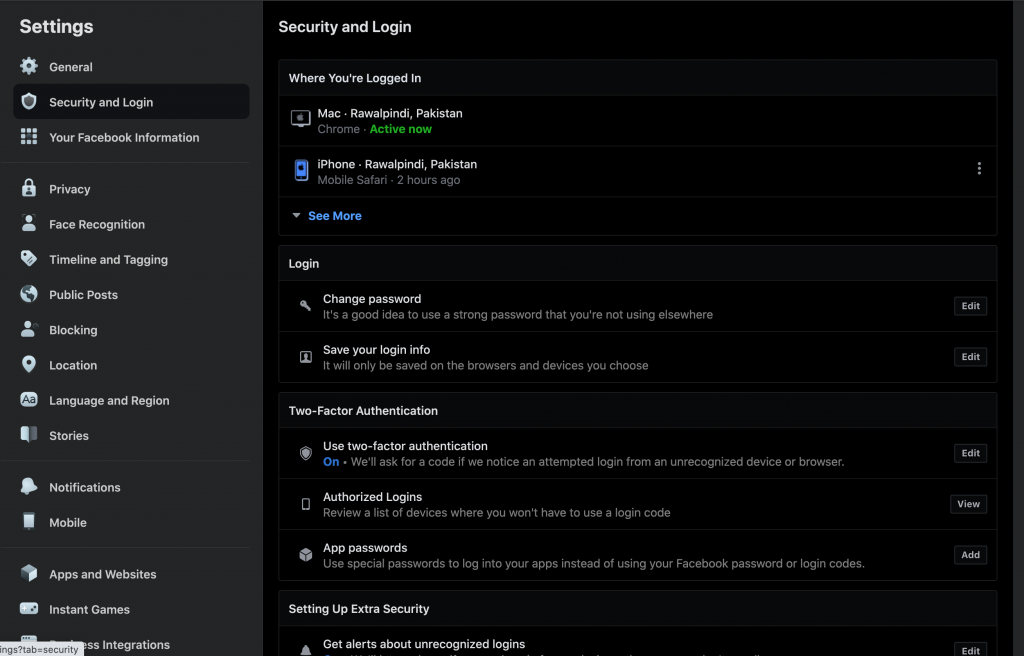Screenshot of an iPhone display showing the Facebook application settings page. The background is black, with the "Settings" and "General" options highlighted in black within the list. The screen further lists various settings categories including "Security and Login," "Your Facebook Information," "Privacy," "Face Recognition," "Timeline and Tagging," "Public Posts," "Blocking," "Location," "Language and Region," "Stories," "Notifications," "Mobile," "Apps and Websites," and "Instant Games."

The "Security and Login" section is expanded, showing multiple sub-options. Under "Where You're Logged In," there's an active session denoted by a green indicator. "Seymour," highlighted in blue, appears next to an icon of three vertical dots, indicating additional settings options. The section includes options such as "Login," "Change Password," and a "Save Your Login Info" setting within a rectangular button labeled "Edit."

Further down, the "Two-Factor Authentication" section indicates that this feature is turned on, with an "Edit" button available. The "Authorized Logins" section has a "View" button within a rectangular box. Another section for "App Passwords" includes an "Add" button, also in a rectangular box.